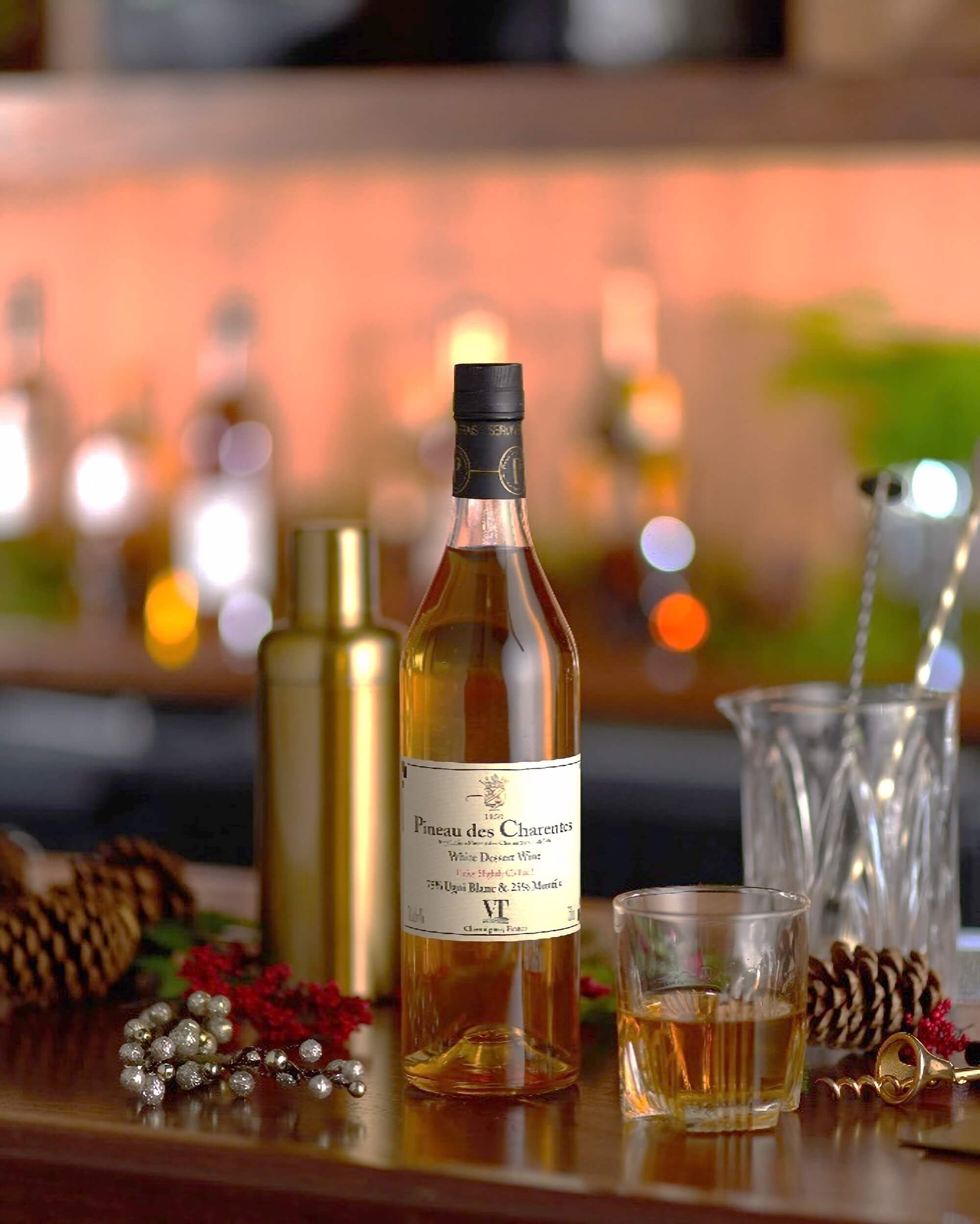This detailed image captures the warm atmosphere of a bar, showcasing a close-up of a wooden bar surface. Dominating the center is a bottle of Pinot de Charentes white dessert wine, characterized by its golden hue and adorned with a white label featuring black text, including "VT" at the bottom. The bottle sports a black top. To the right of this bottle is a small glass, filled halfway with the same golden wine. Scattered around on the bar are a few pine cones—two on the left side of the bottle and one to the right—complemented by silver beads. The upper half of the image blurs into the background, hinting at more bottles of liquor that add to the bar's inviting ambiance. Also, near the right pine cone is a corkscrew bottle opener, and behind the wine bottle, there is a larger cup with mixers and swivel sticks.